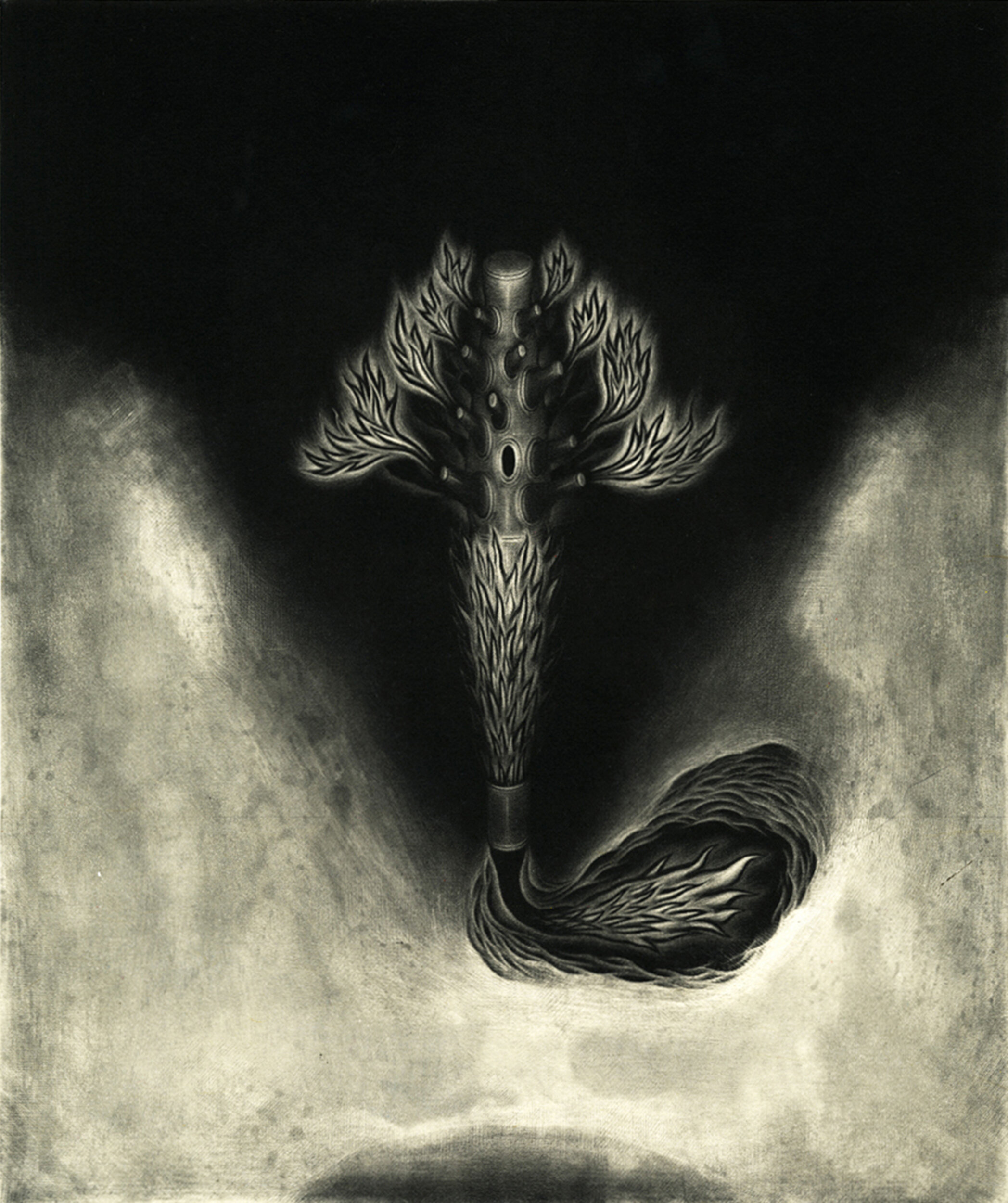In this image, a striking contrast of black, white, and grayish tones forms a dynamic composition. The top half is dominated by an intense black background that melds seamlessly into a gradient of white, gray, and faint tan shades towards the bottom, creating a V-shaped illumination at the center. This lighting focuses on a mystical, cylindrical object that exudes an aura of power and omnipresence. The object, seemingly metallic at the top, features oblong holes and is encircled by symmetrical, upward-bending leaf-like extensions, five on each side, reminiscent of wings or feathers. These feather-like appendages, smaller at the top and elongating as they descend, lend the object an ethereal, feathery appearance. The middle section appears to be wrapped in fur, and at its base, a metallic strip with a tail-like extension swoops gracefully to the right. The entire image, seemingly hand-drawn, blends shades and textures to highlight the mystical object against its dark backdrop, evoking a sense of otherworldly mystery and complexity.